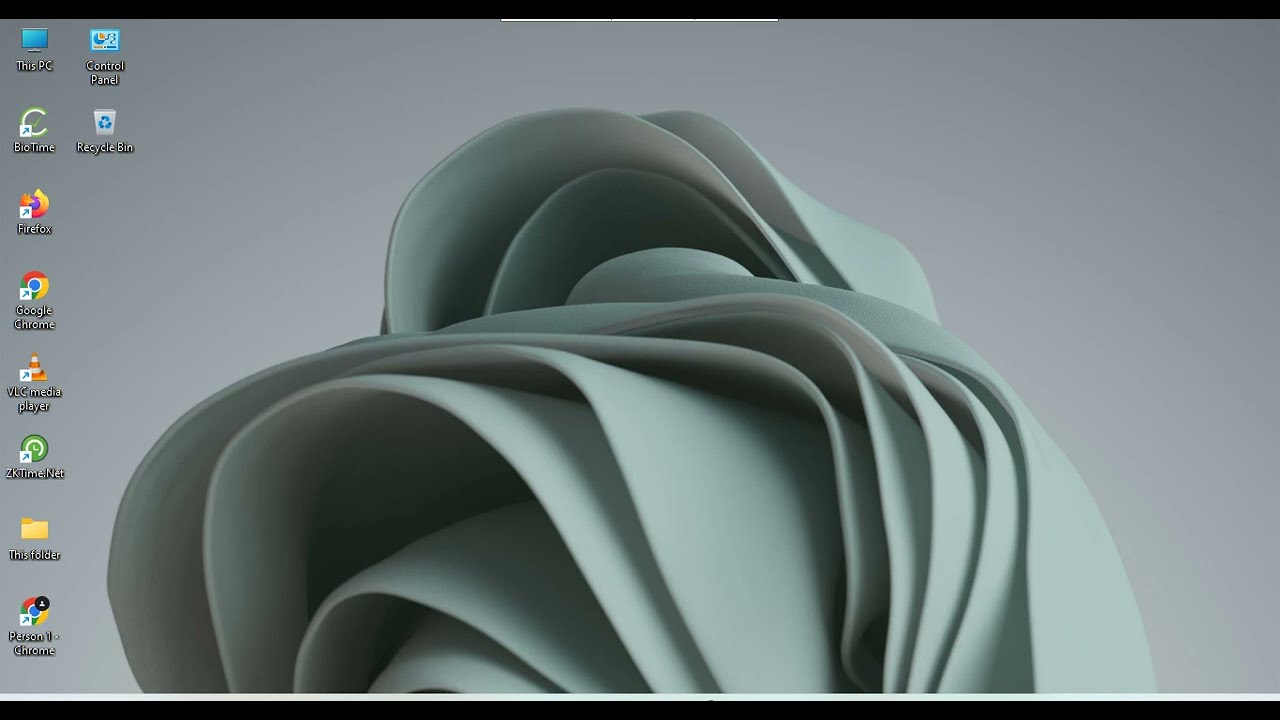The image displays a screenshot of a computer desktop with a unique background and various icons lined up on the left side. The background features a grayscale, zoomed-in image that resembles the intricate layers of a rose, perhaps even evoking thoughts of layered pastries or artistic fabric. The dominant gray tones add to the abstract, detailed design that occupies the center of the screen. 

On the left, the icons are organized into a neat column, starting with 'This PC' followed by 'Biotime,' 'Firefox,' 'Google Chrome,' 'VLC Media Player,' 'zxtime.net,' 'This Folder,' 'Person 1,' and 'Control Panel'. The 'Recycle Bin' icon is situated further to the right, breaking the linear arrangement slightly. There is no visible bottom toolbar, emphasizing the central floral-like imagery and the orderly list of accessible applications and folders.